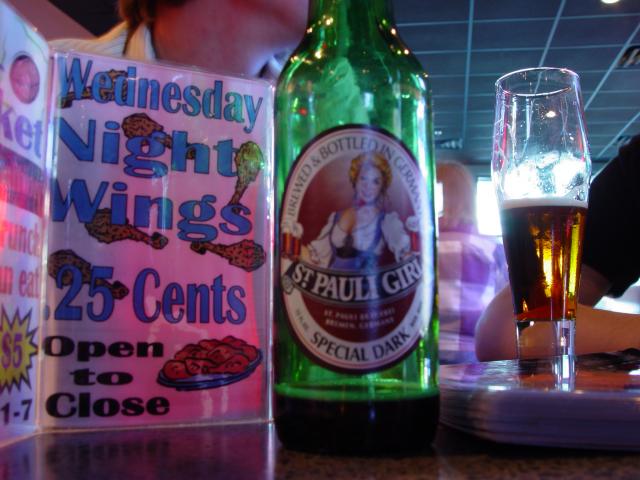The close-up image captures a lively bar scene, focusing predominantly on an eye-catching advertisement promoting "Wednesday Night Wings, 25 cents, open to close," with the text in blue and imagery of wings accompanying it. Dominating the foreground is a green bottle of St. Pauly Girl Special Dark, brewed and bottled in Germany, standing next to a schooner half-filled with beer. The setting includes a wooden table and the high casual atmosphere of the bar, punctuated by visible elements like a flannel shirt and the backs of patrons, suggesting a busy and social environment. Although the faces are obscured, several people are discernible, with one person's elbows resting on the bar and another's neck in the foreground, giving the scene a sense of intimate camaraderie and typical barroom chatter. The backdrop hints at a bright yet cozy ambiance, despite the bar’s slightly worn-in look.